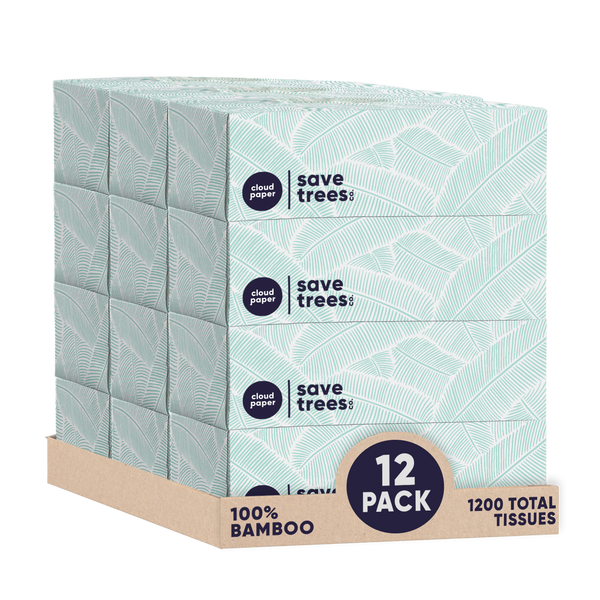This highly detailed photograph showcases an advertisement for a bulk pack of tissues, ideal for online shopping. The background is stark white, making the product stand out prominently. At the forefront is a large, eco-friendly, brown cardboard box holding 12 smaller rectangular tissue boxes arranged in a 3x4 stack. Each individual tissue box is a light green color, adorned with an intricate leaf pattern that resembles green and blue fern leaves, reflecting an organic, nature-inspired design. Prominently displayed on the top-left corner of each tissue box is the phrase "Save Trees" in notable black text, underscoring the product's eco-conscious theme.

The main box features a striking blue circle that boldly announces "12 Pack." Below this, additional key details are listed: "100% Bamboo" on the left, emphasizing the sustainable nature of the tissues, and "1200 Total Tissues" on the right, highlighting the quantity provided. The overall packaging design not only emphasizes the product's environmental benefits but also its practicality and generous supply, making it a compelling choice for conscious consumers.